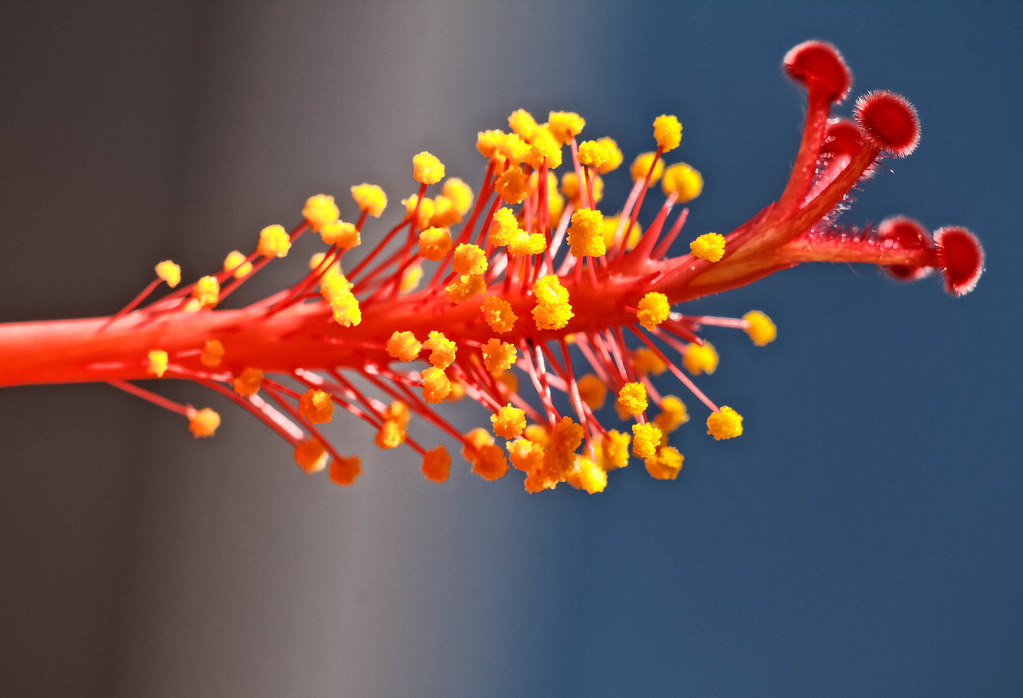This professionally captured close-up image showcases an unusual plant with striking details. Dominating the center of the composition is a thick, vivid cherry-red stem that extends horizontally from the left. Along this primary stem, there are numerous smaller offshoots, each bearing clusters of puffy yellow structures, resembling pollen or tiny flowers, meticulously arranged and vividly in focus. The red stem culminates in several mushroom-shaped caps or furry orbs, adding an intriguing texture to the plant. The background is a softly blurred gradient of gray, light white, and blue, enhancing the plant's vibrant colors. This visually arresting photograph, void of any text, is conspicuous for its precision and professional quality, likely achieved with a specialized, high-end camera.